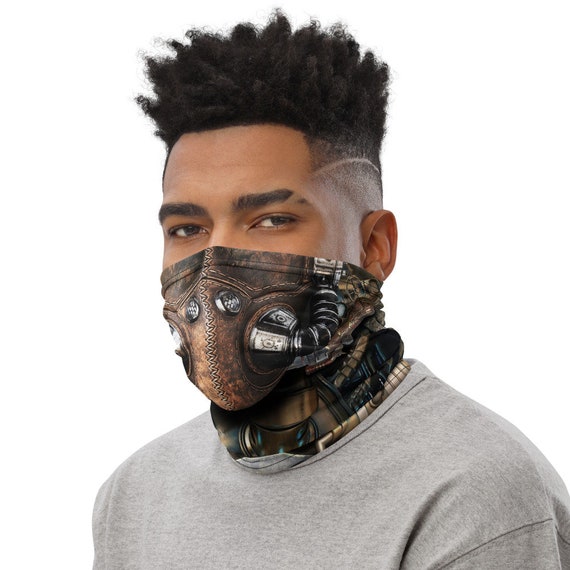This image is a detailed portrait of a man of African descent with dark skin, showcased against a plain white background. He stands out due to his direct and intense gaze at the camera. His hair is meticulously groomed, featuring a poofy, curled top that contrasts with a tightly faded lower section. A distinct scar cuts through his left eyebrow, creating a slit that continues into his hairline. He is adorned in a gray crew neck shirt and wears a distinctive bandana that covers the lower half of his face, up to his nose. The bandana has a rustic, steampunk design, featuring metal pipes extending from either side of his mouth, resembling a gas mask's apparatus. Stainless steel cogs and piping imagery ascend from the mask, covering his neck and adding a metallic, industrial aesthetic to his appearance.